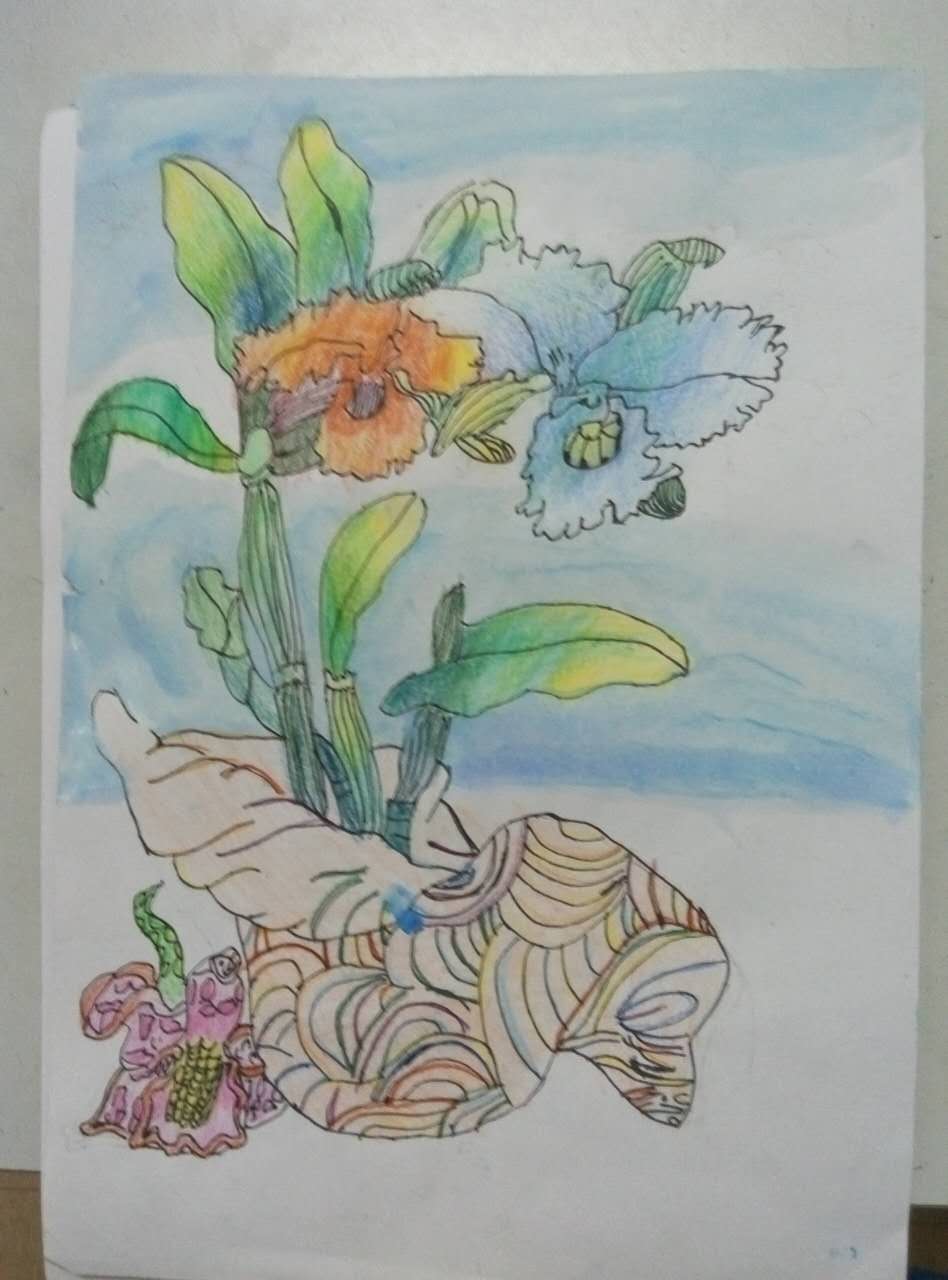This is a photo of a detailed, hand-drawn illustration on a large, rectangular sheet of white paper. The central focus of the drawing is an ornate, colorful seashell with numerous parallel curving lines and vibrant swirls of yellow, blue, and orange. Emerging from the seashell are three distinct stalks adorned with flowers and leaves. One stalk holds an orange and a blue orchid with large green leaves shaded yellow at the tips, while another has a lone bud about to blossom. A third stalk bears only a large leaf. Lying beside the seashell is a pink orchid flower with a yellow corncob-textured center and a waving stem. The top part of the background is shaded blue, resembling either a sky or water, while the lower portion remains the untouched white of the paper. This intricate and colorful illustration exudes the charm of an adult coloring book.